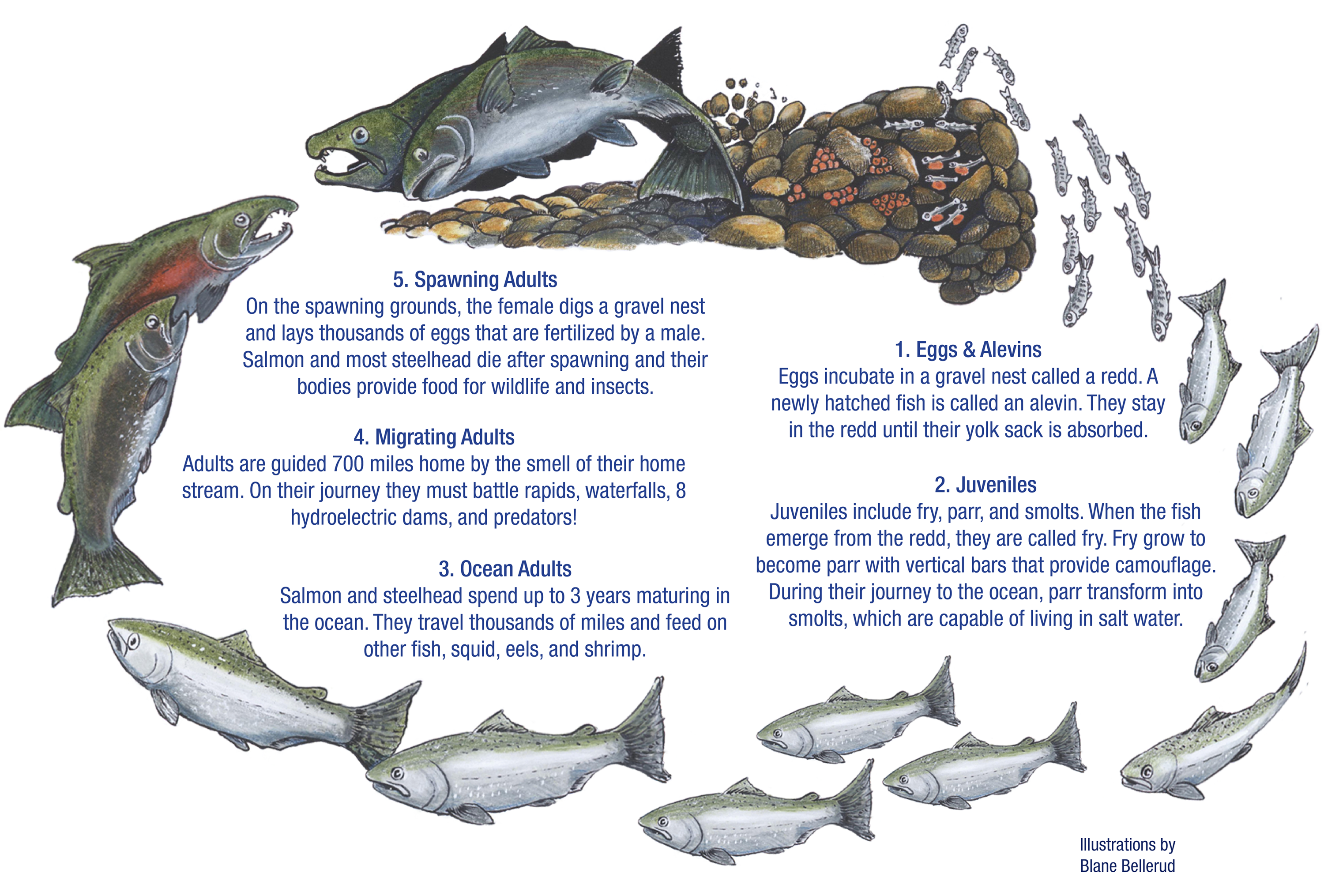This hand-drawn illustration vividly depicts the life cycle of a salmon, encircled by detailed text describing each stage. Starting at the top, you see a cluster of rocks with eggs hatching. Moving clockwise, the fish's progression from tiny babies to fully grown adults is illustrated. In the center, five key stages are labeled: "One, Eggs and Alvens," "Two, Juveniles," "Three, Ocean Adults," "Four, Migrating Adults," and "Five, Spawning Adults." Each label includes a detailed paragraph describing the salmon's life at that stage. The illustration culminates in the lower-left corner, showing adult salmon laying eggs, completing the cycle. Notably, at the bottom right corner, it is annotated with, "Illustrations by Blaine Bellarude." The detailed text and vibrant drawings work together to provide a comprehensive and educational overview of the salmon's lifecycle.